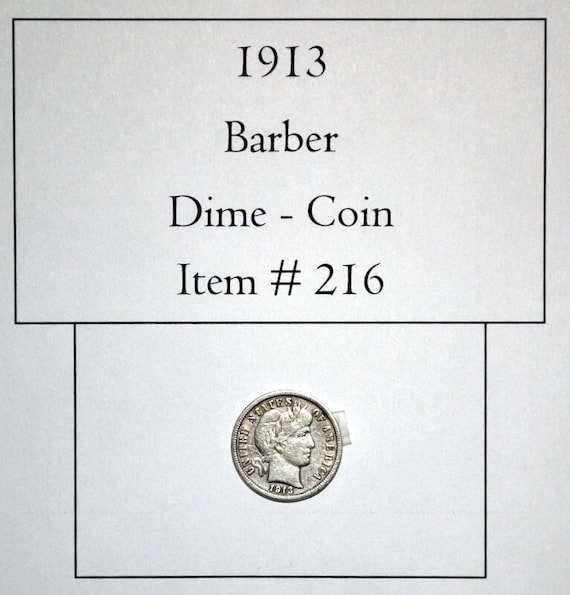The image features a cardboard display with two distinct sections. The top section is a rectangular box that prominently displays text in black letters, reading "1913 Barber Dime Coin, Item Number 216." Below this, a slightly shorter rectangular section is perfectly aligned and centered. This lower section houses a 1913 Barber Dime, taped securely with cellophane tape. The coin itself is silver-colored and showcases a right-facing profile of a man with short hair. Arched around his head are the words "United States of America," with the year "1913" also inscribed. The background of the display is a light gray, giving it a clean and straightforward presentation suitable for stacking or selling.